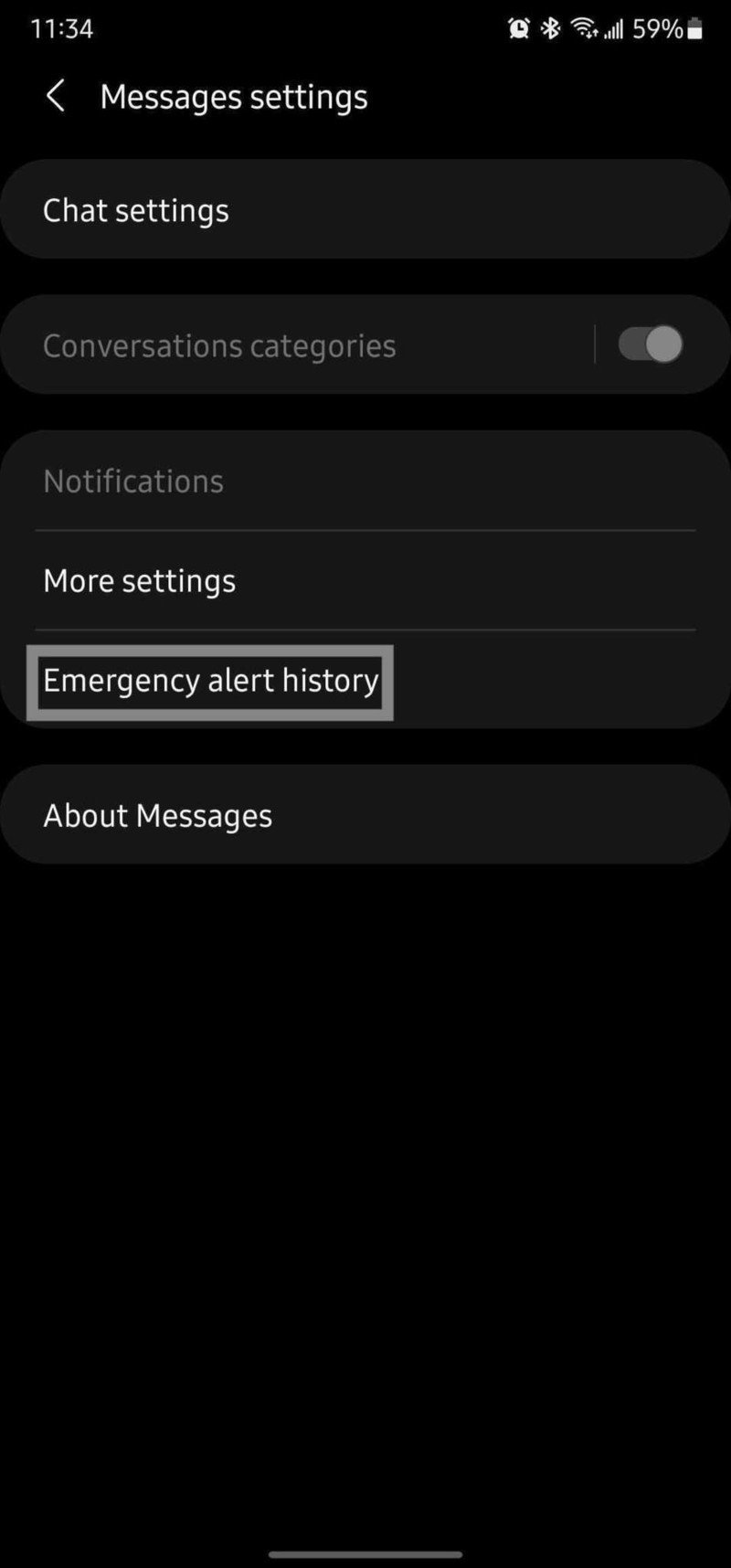**Caption:**

A detailed screenshot of a smartphone using dark mode. The top section displays the time "11:34" in white text against the dark background, with icons indicating alarm clock, Bluetooth, full Wi-Fi, full signal strength, and a battery at 59% capacity. Below this, an arrow pointing left indicates a "Back" action. The interface shows "Messages Settings" as the main heading, followed by "Chat Settings." A grayed-out "Conversations Categories" section features a slider that is positioned to the right but remains inactive. Further down, in gray text, "Notifications" is noted, followed by "More Settings" in white text with a blue highlight. A large gray box encases the "Emergency Alert History" option. At the bottom, "About Messages" is listed. A vertical gray slider for navigation is present at the center-bottom of the screen. The description indicates no further content beyond these elements.